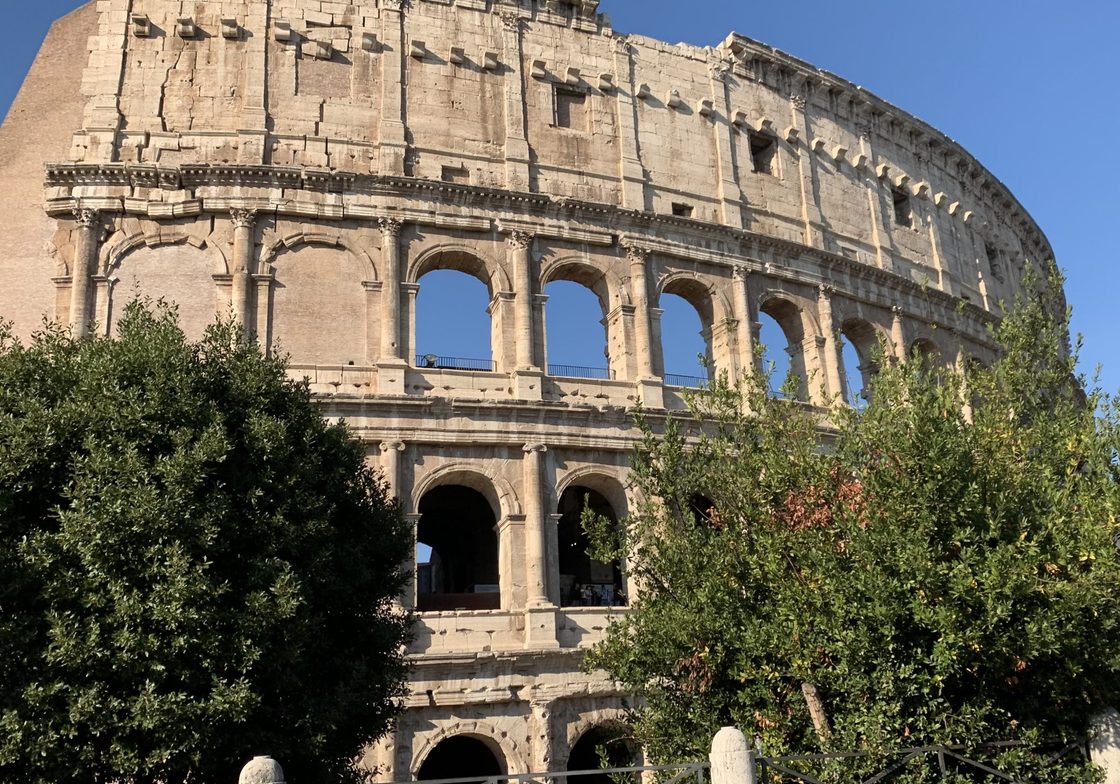The photograph captures a detailed section of an ancient, light brown coliseum, possibly the Roman Colosseum. The towering structure is four stories high. The first three floors feature large open arches, revealing a mix of dark interiors and open sky. The fourth, uppermost floor has solid walls adorned with decorative trim and square openings that may have once been windows. The top trim line of the coliseum is partially crumbled, evidencing its age and wear.

The scene is set outdoors on a cloudless day, with a vibrant blue sky framing the ancient edifice. Flanking the coliseum's base are two bushes: one lush and fluffy, the other noticeably scrawnier. A fence with white poles and black metal fins runs along the bottom of the image, indicating that the structure is likely enclosed for preservation or visitor safety. The composition suggests a glimpse into a timeless architectural marvel, now encased in nature and modern boundaries.